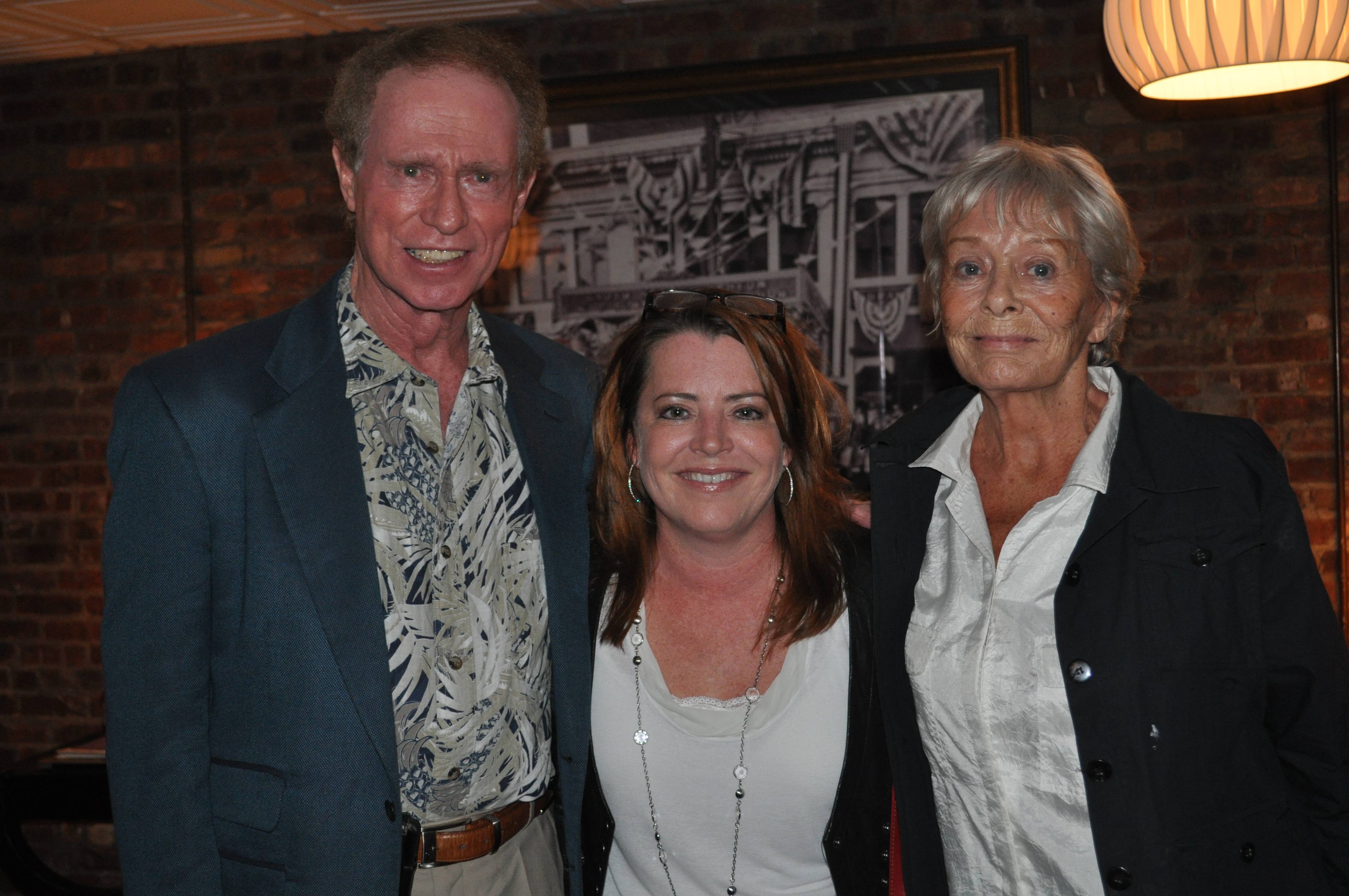This photograph features three individuals posing closely together, each with their arms wrapped around one another, all smiling. In the background is a red brick wall adorned with a large black-and-white framed picture of a building decorated with numerous flags, hinting at a historical or patriotic moment. To the upper right of the image hangs a round light fixture, while the top left reveals a section of a white drop-down ceiling.

On the left stands an older man, likely in his late 50s or early 60s, with grayish-red hair. He is dressed in khaki pants paired with a light brown leather belt with a silver buckle, a blue sports jacket, and a Hawaiian-style gray and white button-up shirt.

The central figure, a woman probably in her late 30s or early 40s, sports a white blouse with a long silver necklace that extends beyond the frame. She has shoulder-length reddish-brown hair and wears hoop earrings, along with glasses perched on top of her head.

On the right is an older woman, likely in her 60s, with short gray hair above her ears. She is clad in a black coat over a white button-up shirt.

The image captures a warm, shared moment against a rich backdrop of historical and architectural details.